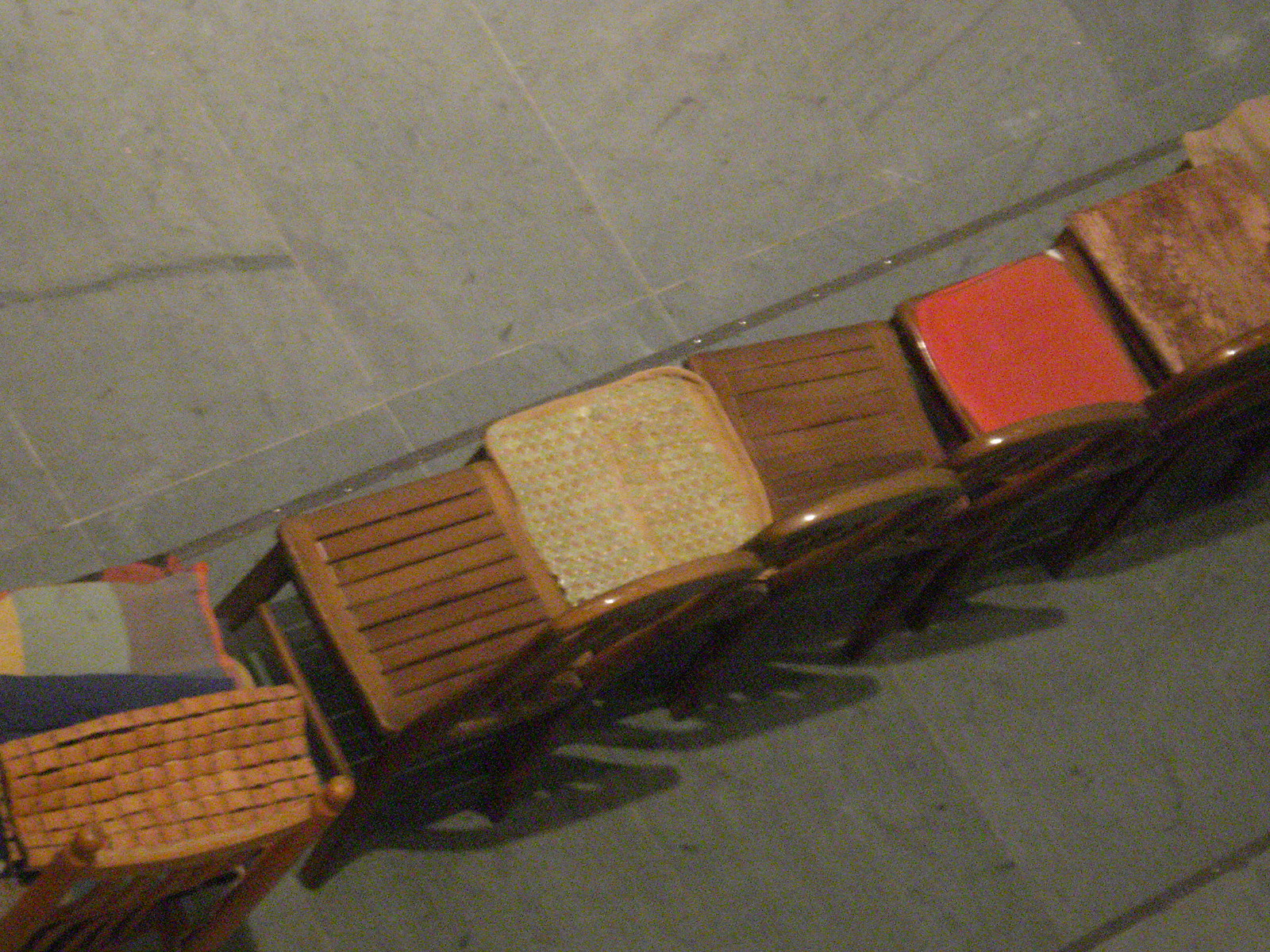This is a color aerial photograph capturing a row of seven distinct chairs placed side by side on a grayish tile floor with noticeable caulking between the tiles. Each chair is unique in design: one has wooden slats for the seat, another features a wicker bottom, one boasts a red cushion, and yet another has a solid, slightly worn wooden seat. Some backs of the chairs cast shadows on the floor, adding depth to the image. Additionally, there is a chair with a yellow cushion and another that might have a plaid throw blanket draped over a potentially broken backing. The rounded dark brown wood backs of the chairs further add to their uniqueness. The setting remains unidentified, as no text in the photograph indicates whether it is in a restaurant or another location.